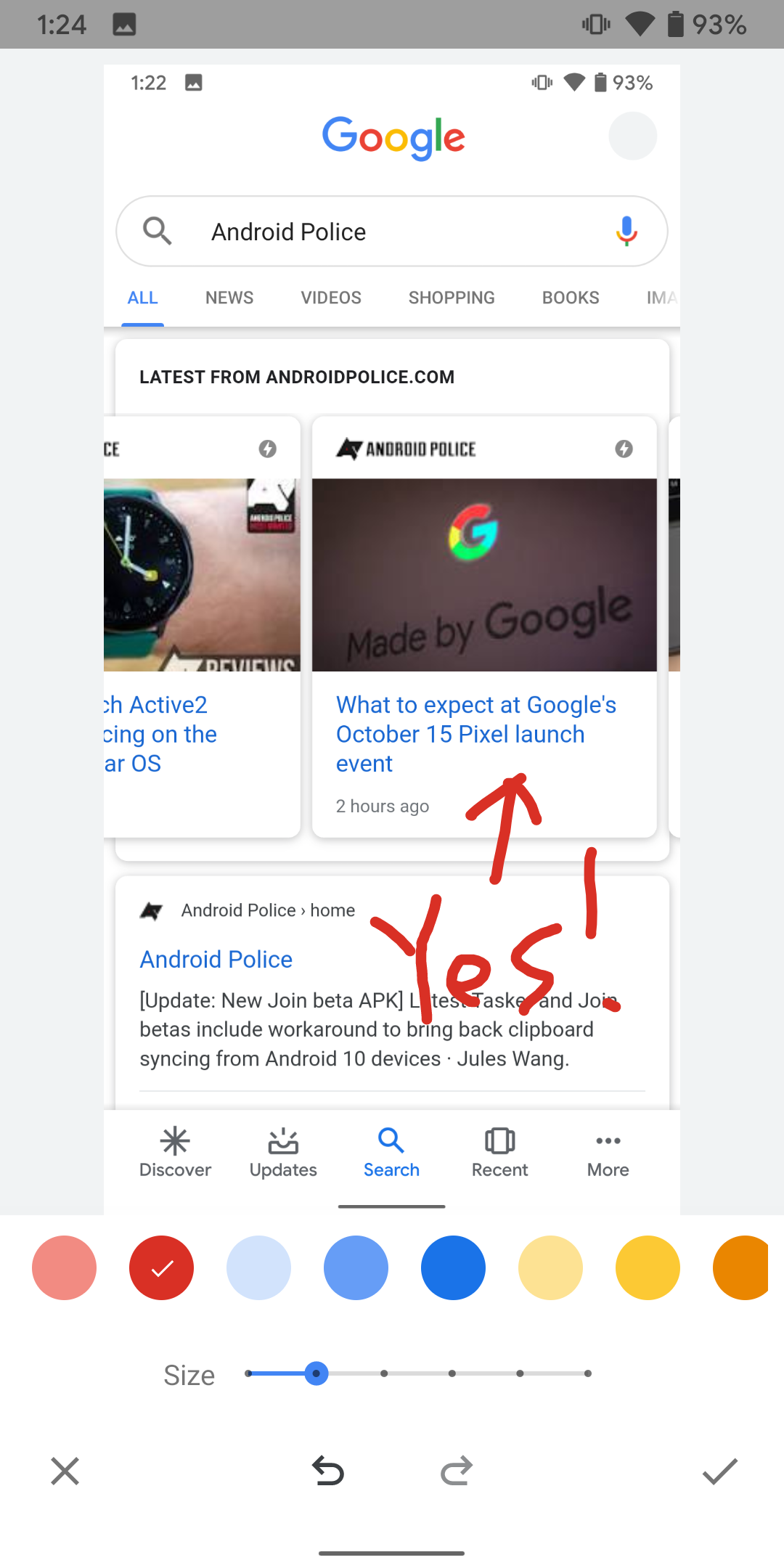This image is a screenshot taken from a mobile device, though it is unclear whether it is an Android or iOS device. The navigation bar at the bottom of the screen is distinctive, featuring a cross (X) icon on the lower left, a back button in the center, a forward button next to it, and a check mark icon on the lower right.

The screenshot displays a Google search page, with the query "Android police." The screen shows a search result titled "Latest from Android Police," featuring an article with the Google logo and the headline: "What to expect at Google's October 15th Pixel launch event." Overlaid on this result is the text "YES!" in uppercase, written in red, accompanied by a red arrow pointing toward the article headline.

At the very bottom of the image, a red color selection is visible, indicating that the overlay text and arrow were recently added using an editing tool before the screenshot was taken. The buttons at the bottom likely belong to this editing interface, providing options to undo (X button), navigate through edits (back and forward buttons), and confirm changes (check mark button).